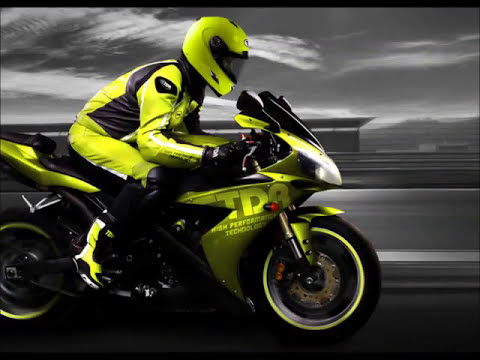The image depicts a man riding a bright yellow and black motorcycle, speeding down a highway. He is clad in a matching yellow and black motorcycle bodysuit, with a similarly colored helmet. The motorcycle features the letters "TDR" and the phrase "high performance technology" on its side. Notably, the background is in black and white, showcasing a blurred roadside and a gray sky with white clouds, emphasizing the motion and speed of the scene. The man and the motorcycle are the only elements in color, drawing attention to the vivid yellow against the monochromatic backdrop.